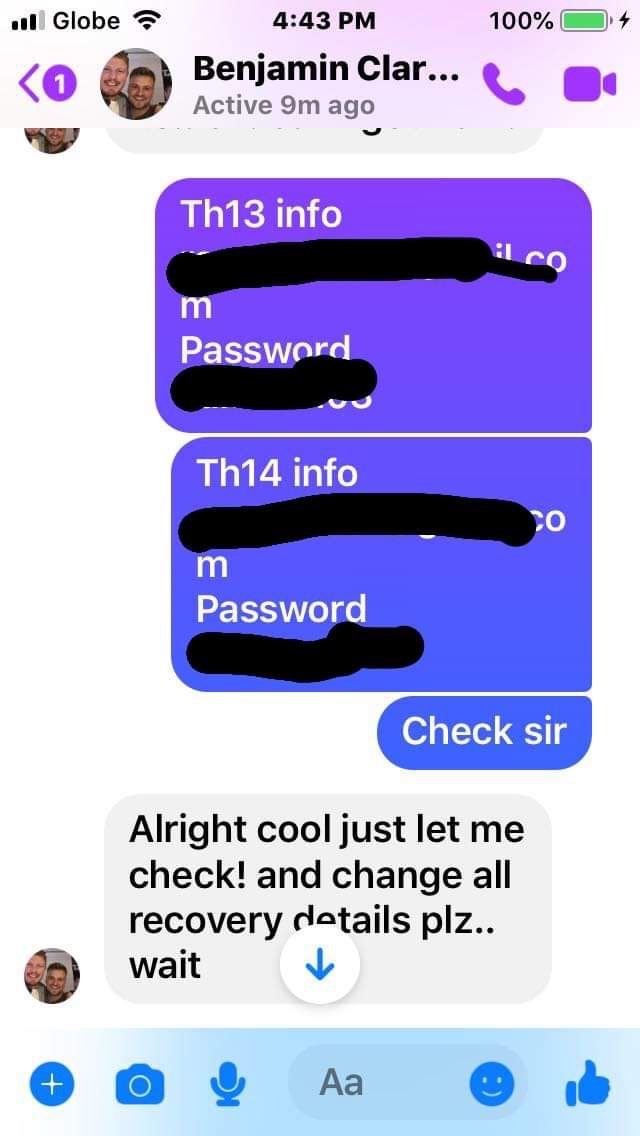This image is a screenshot of a social media reply or messaging interface on a smartphone. The screen shows a conversation with Benjamin Clare, whose profile picture is partially concealed, with only the letters "C-L-A-R" visible. The message from Benjamin Clare indicates he was active 9 minutes ago. In the top-left corner, a back button is visible, alongside a notification icon featuring a white number one within a purple circle. The top-right corner indicates the phone's signal strength under the carrier "Globe," showing a full 100% battery level at 4:43 PM.

The conversation contains sensitive information that has been redacted. It mentions "TH13 info" and "TH14 info" followed by a partially hidden letter 'M' and the word 'password,' with both the website and password obscured by black scribbles. Benjamin’s response reads: "Alright cool just let me check and change all the recovery details, please wait." The primary colors in this interface are white, black, and blue, and the screen also has icons for phone and camera functionalities, emblematic of the messaging or social media platform.